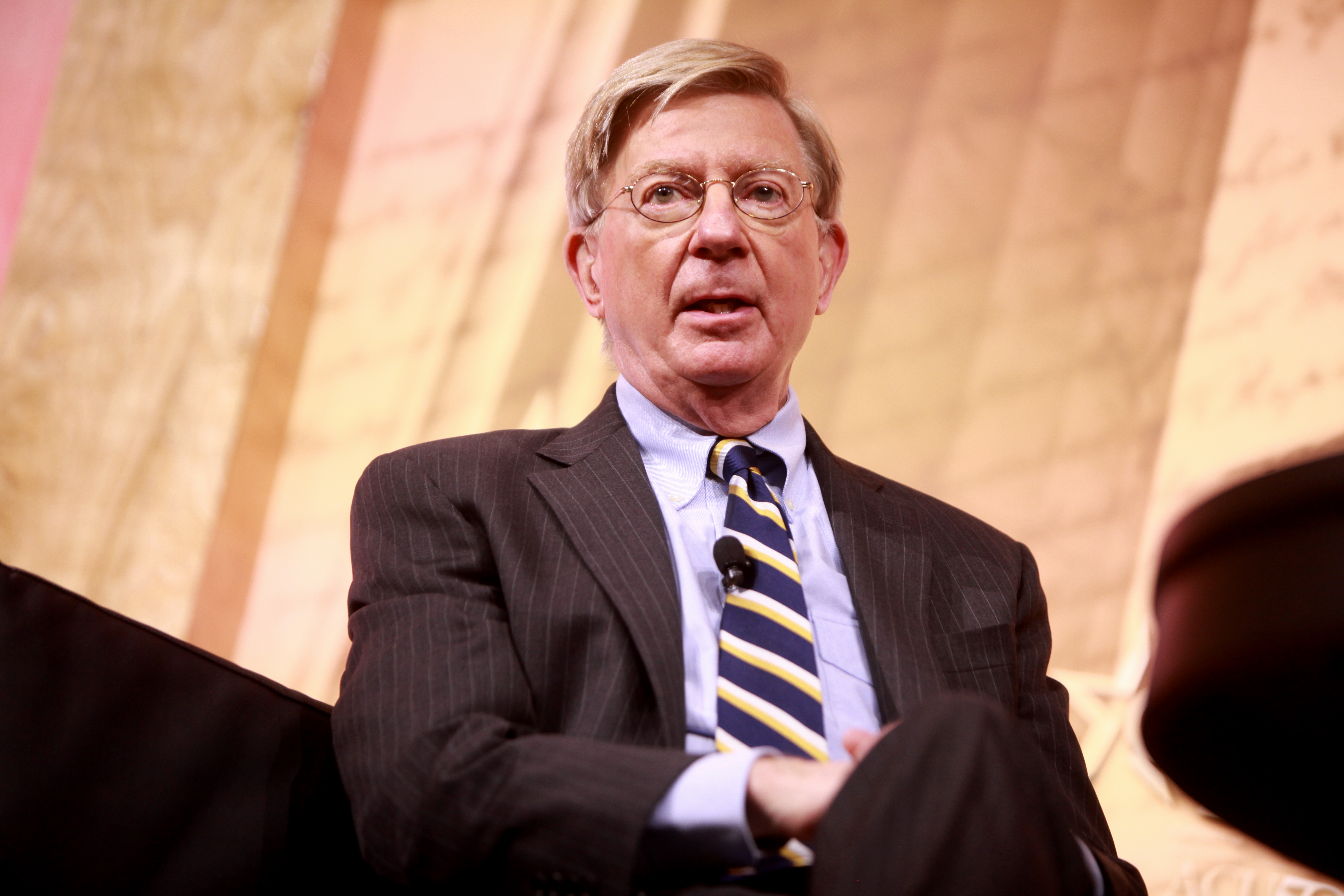The photograph portrays a close-up of an older Caucasian man, probably in his 60s or 70s, who appears to be a politician. He has a clean-shaven face marked by numerous wrinkles and notable dimples beside his nose and mouth. His hair, which seems to have been blonde in his youth, now shows signs of gray, particularly around the temples, and appears either dyed back to blonde or possibly a wig. He wears wire-rimmed round glasses perched on a long nose bridge.

Clad in a dark gray pinstripe suit with light gray stripes, he is also wearing a light blue collared dress shirt. A navy blue necktie with white and yellow diagonal stripes is fastened to his chest, adorned with a small clipped-on microphone, suggesting he is mid-discourse. The man is seated, with the image showing him from the waist up, including part of his knee. The background features a tan grid pattern with varying shades of light and dark tan, adding to the visual depth of the setting.